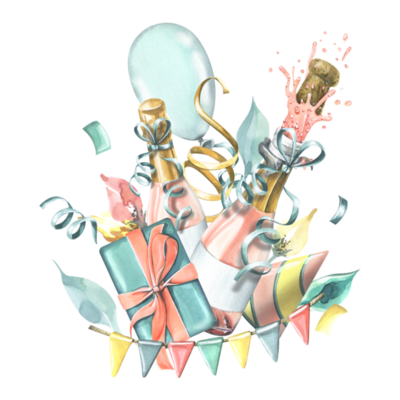This image depicts a festive party scene against a white background, centered around a green gift box adorned with a pink ribbon and flanked by various vivid party elements. Dominating the middle of the image, there is a bottle of champagne spraying pink liquid upwards, creating the impression of celebration. A similar champagne bottle, this one closed with a blue ribbon, appears at another point in the scene. The background is brightened with a green balloon floating near the top middle and colorful, cone-shaped party hats in yellow and pink scattered around. The picture further bursts with energy through a garland of triangular pennant flags in a repeating pattern of yellow, blue, red, and green, stretching across the scene. Accentuating the festive theme, flashes of blue confetti and yellow swirls on the pink cones add a vibrant touch to the overall composition, capturing the essence of a lively, joy-filled party.